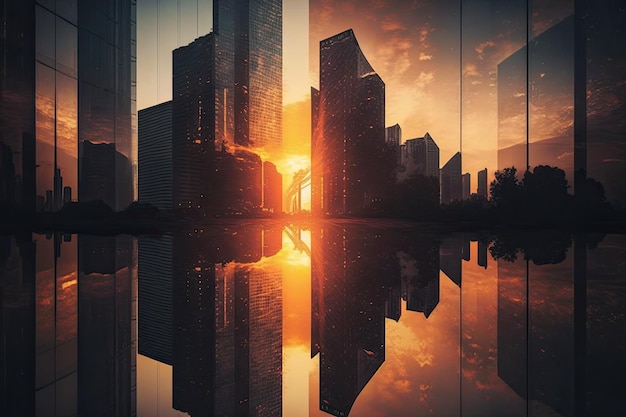This rectangular photograph, approximately 4 inches wide and 3 inches high, captures a striking urban scene dominated by tall, modern skyscrapers with numerous windows. The image is bisected horizontally, with the lower half serving as a mirror-like reflection of the top half, as if on a still, reflective water surface or a reflective glass. The upper portion features a city skyline bathed in the soft light of either sunrise or sunset, creating an orange hue that highlights some of the buildings and clouds in the blue sky. Among the towering structures, a notable gap reveals a sliver of the vibrant orange sun illuminating white and orange clouds. Distinct color variations appear, with some buildings reflecting a bluish light in their windows, while others display a more pronounced orange glow. On the right hand side of the lower half, trees or bushes are visible, adding a touch of natural greenery to this urban landscape. Overall, the composition creates a symmetrical, almost surreal scene with the tranquil reflection perfectly mirroring the cityscape above.